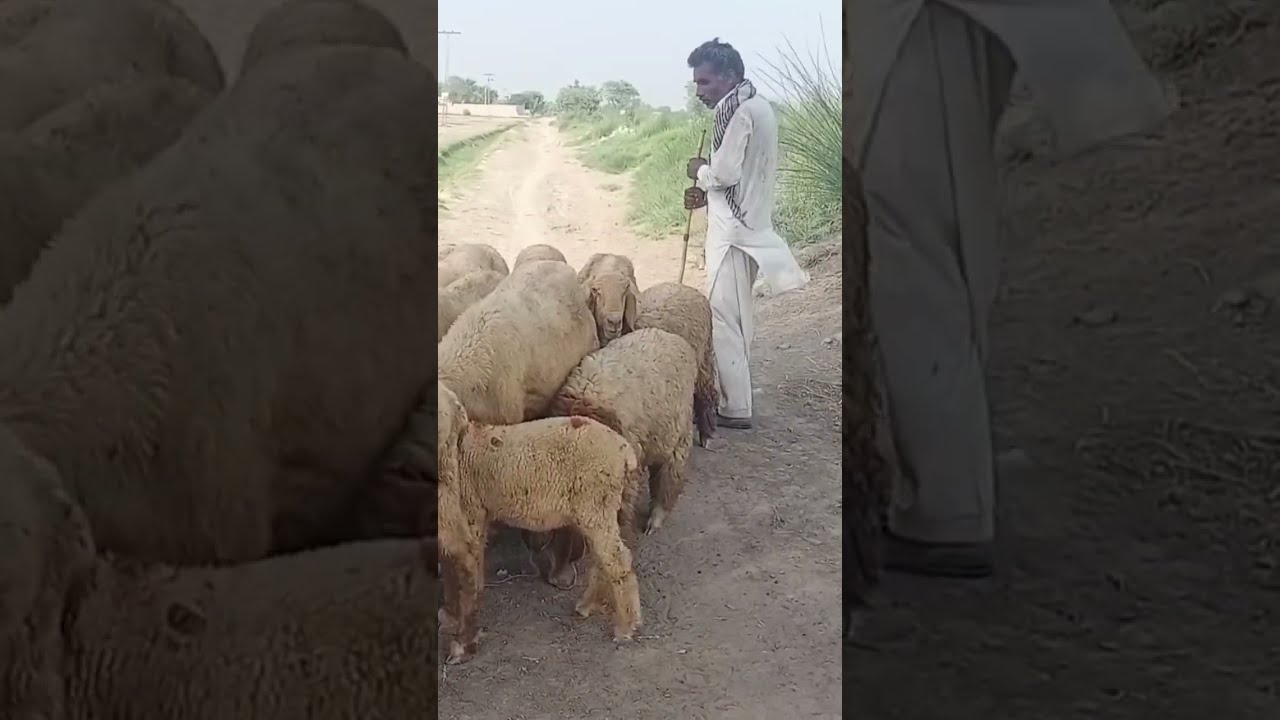This photograph, set in an Indian village, depicts a lean and fit man herding sheep along a dirt road. The man, with dark skin and black hair, is dressed in traditional, casual Indian attire consisting of a white long-sleeve shirt and white pants. He holds a wooden pole firmly in both hands. The flock of sheep huddles around him, some standing and others walking, while green shrubs and grasses flank the dirt road on either side.

The central image, shaped like a smartphone screen—taller than it is wide—is brightly lit and rendered in vivid detail. This primary photograph is bordered by faded, darkened segments of the same scene that extend to the sides, creating a frame. On the left, there is a close-up of the sheep, and on the right, a close-up of the man's legs. These surrounding areas serve as a transparent, shaded backdrop, enhancing the focus on the central scene.